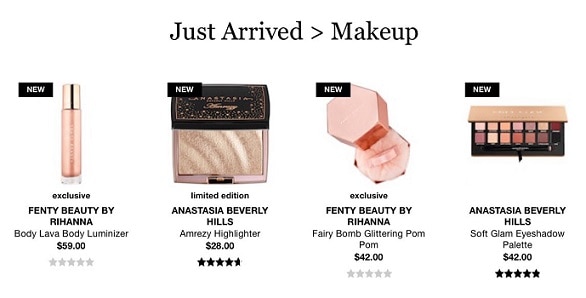Here are four new makeup products that have just arrived:

1. **Fenty Beauty by Rihanna Body Lava Body Luminizer**: This exclusive lip gloss features a sleek design with the word "exclusive" prominently displayed. Priced at $59, this body luminizer currently has no reviews. The packaging includes a white label with a black box announcing its novelty.

2. **Anastasia Beverly Hills Amrezy Highlighter**: This new highlighter costs $28 and has a rating of 4.5 out of 5 stars. The product stands out with a shimmering finish, perfect for adding a radiant glow to your makeup routine.

3. **Fenty Beauty by Rihanna Fairy Bomb Glittering Pom Pom**: Another exclusive from Fenty Beauty, this glittering pom pom is priced at $42. Like the Body Lava, it currently has no reviews. The product promises a fun and unique way to apply glitter to your skin.

4. **Anastasia Beverly Hills Soft Glam Eyeshadow Palette**: This highly-rated eyeshadow palette, with a perfect 5-star rating, retails for $42. The palette features a range of rose gold and brown hues, making it ideal for creating soft, glamorous looks.

These newly launched items are displayed on a white background, with each product depicted in full color. The prominent "Just Arrived in Makeup" title is featured in bold, black font, with a right arrow indicating the latest additions.